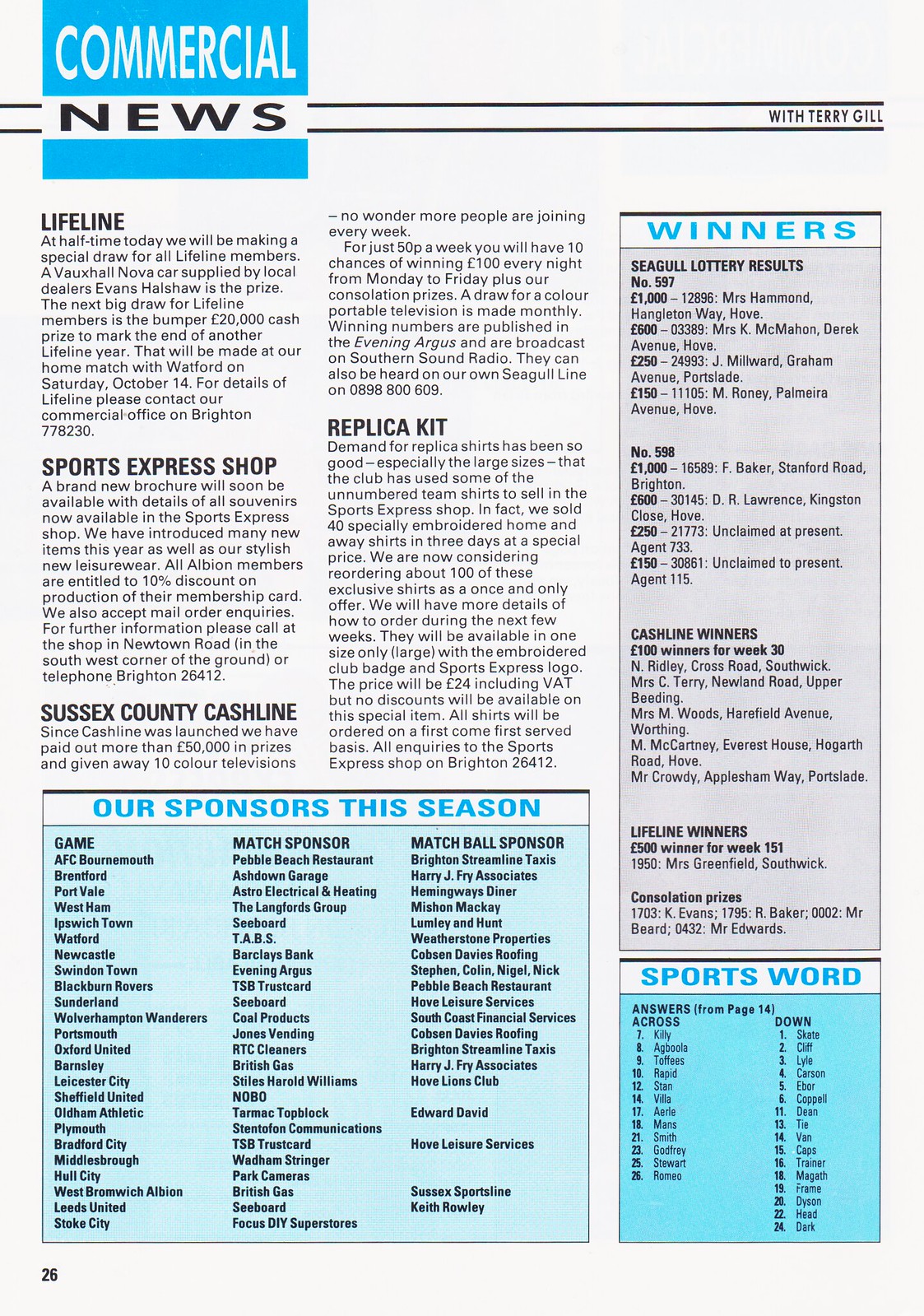This image appears to be a page from a periodical, specifically a sports program. At the top left, prominently displayed in white letters on a blue background, is the title "Commercial News," followed by "With Terry Gill" on the right. The page is divided into three main columns, each containing various sections.

The first column begins with a section titled "Lifeline," which mentions a special draw for all Lifeline members. Beneath this is another section labeled "Sports Express Shop," announcing an upcoming brochure detailing the souvenirs available. The final section in this column is "Sussex County Cash Line," highlighting that over 50,000 pounds have been paid out in prizes and ten color televisions given away since its launch.

In the second column, the "Sussex County Cash Line" section continues briefly before transitioning to a section called "Replica Kit." Here, it is noted that the demand for replica shirts, especially in large sizes, has been so high that the club has had to sell unnumbered team shirts in the Sports Express Shop. Below this, there is a blue rectangle with white text listing "Our Sponsors This Season."

The third column on the right side features a title "Winners" detailing various winners, including those from the Segal Lottery and Lifeline. Underneath this section is "Sports Word," which contains answers to a crossword puzzle, specified as being from page 14.

At the very bottom left of the page, the number 26 is printed, indicating the page number in this sports program.